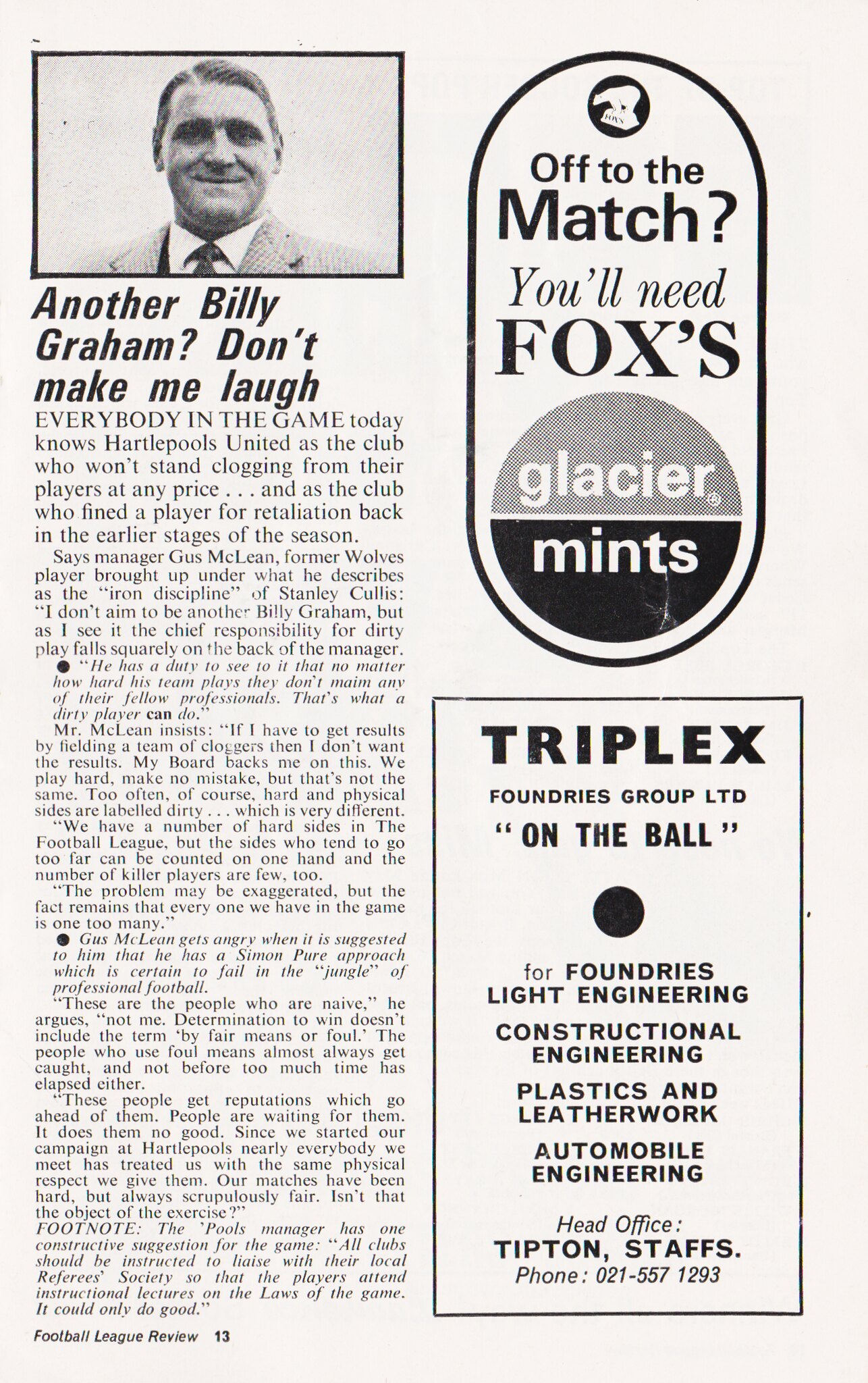The image displays a newspaper clipping set against a light green background. In the upper left corner, there's a black and white photograph of an older man with combed-over hair, wearing a suit and tie. Below this image, a bold heading reads, "Another Billy Graham? Don't make me laugh." This is followed by a long column of text. On the right side of the clipping, there are two advertisements. The top ad, shaped like a pill outline, promotes Fox's Glacier Mints with the tagline, "Off to the match? You'll need Fox's Glacier Mints." Below that, the second ad in a black box reads, "Triplex Foundries Group Limited. On the ball for foundries light engineering, construction engineering, plastics and leatherwork, automobile engineering. Head office: Tipton Staffs. Phone: 021 557 1293." In the bottom left corner of the clipping, in smaller print, it states, "Football League Review 13."